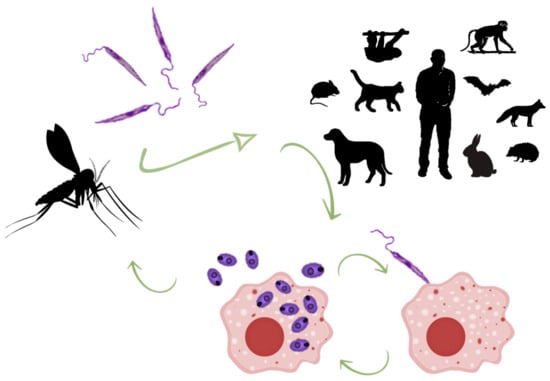The image is an informational poster illustrating the transmission cycle of a mosquito-borne disease. It features a white background and is designed in landscape orientation. On the far left, there's a prominent black silhouette of a mosquito. From the mosquito, a gray arrow points rightward toward various black silhouettes representing creatures that the mosquito can infect, including a man, dog, cat, mouse, rabbit, raccoon, fox, bat, monkey, and tree sloth. Above this arrow, four purple straight lines with squiggly ends represent microorganisms or parasites carried by the mosquito.

Below the sequence of infected hosts, another gray arrow points downward to a pink blob with a red circle at its center, symbolizing a cell infected by the parasite. Purple egg-like shapes are depicted both inside and outside the pink blob, indicating the proliferation of the microorganisms. An additional arrow points rightward to a second pink blob, similar to the first, from which one of the purple lines with squiggles re-emerges to attach to the blob, transforming into purple egg-like structures.

A final sequence of arrows loops the process back to the mosquito, illustrating how the disease propagates through its life cycle and spreads from mosquitoes to humans and other animals. This detailed diagram effectively demonstrates the complex life cycle and transmission path of the disease.